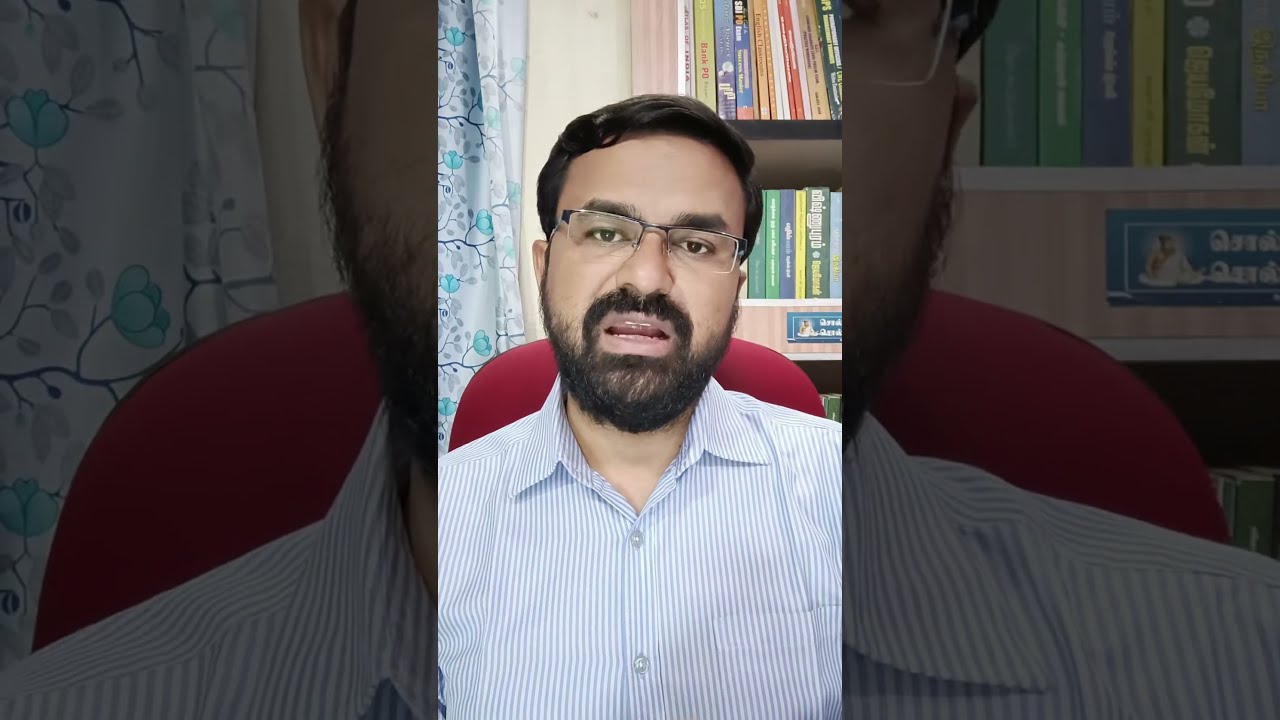The photograph prominently features a man with short black hair, a beard, and a mustache. He's wearing wire-rimmed glasses and a blue and white striped button-down shirt, which is unbuttoned at the collar. His head is tilted slightly to his right, revealing more of his left ear, and his mouth is slightly open, showing some of his upper teeth. The background consists of at least two or three shelves filled with books of various colored bindings, including blue and yellow. 

To the man's left is a red chair, and behind him is a drape and a portion of a beige wall. Additionally, the image has two magnified sections: the right third zooms in on the right half of the man's face and shoulder, and the left third on the left half, making minor details more prominent but slightly blurred. The overall color scheme of the image includes shades of blue, white, and black, with the background appearing somewhat faded compared to the central figure. There is also a small indistinct panel situated beneath the books on the shelves.